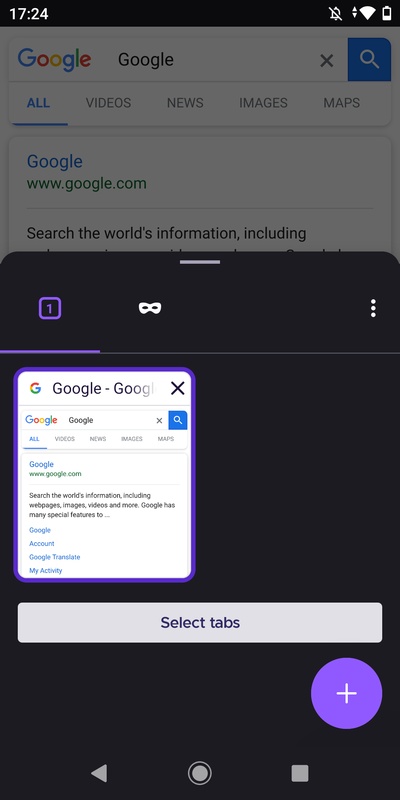The image depicts a smartphone screen showcasing various elements. In the top left corner, the clock displays the time as 17:24 in white numerals. On the right-hand side, there is a notifications icon that appears to be switched off, along with a WiFi signal indicator, and a battery icon indicating a low charge. The background of the screen features a Google search bar, with a dark grey panel superimposed over it. On the left side of the panel is a number one, encased in a purple box and underlined in purple. Below this, there is a miniature version of the same Google search window, depicted as a small rectangle bordered in purple, mirroring the content of the background search. Further down, a large grey tab in the center of the screen reads "Select Tabs" in purple text. To the right of this tab, there is a purple circle with a white plus symbol at its center. At the very bottom of the screen, there are three grey navigation icons: a triangle on the left, a circle within a circle in the middle, and a square on the right.